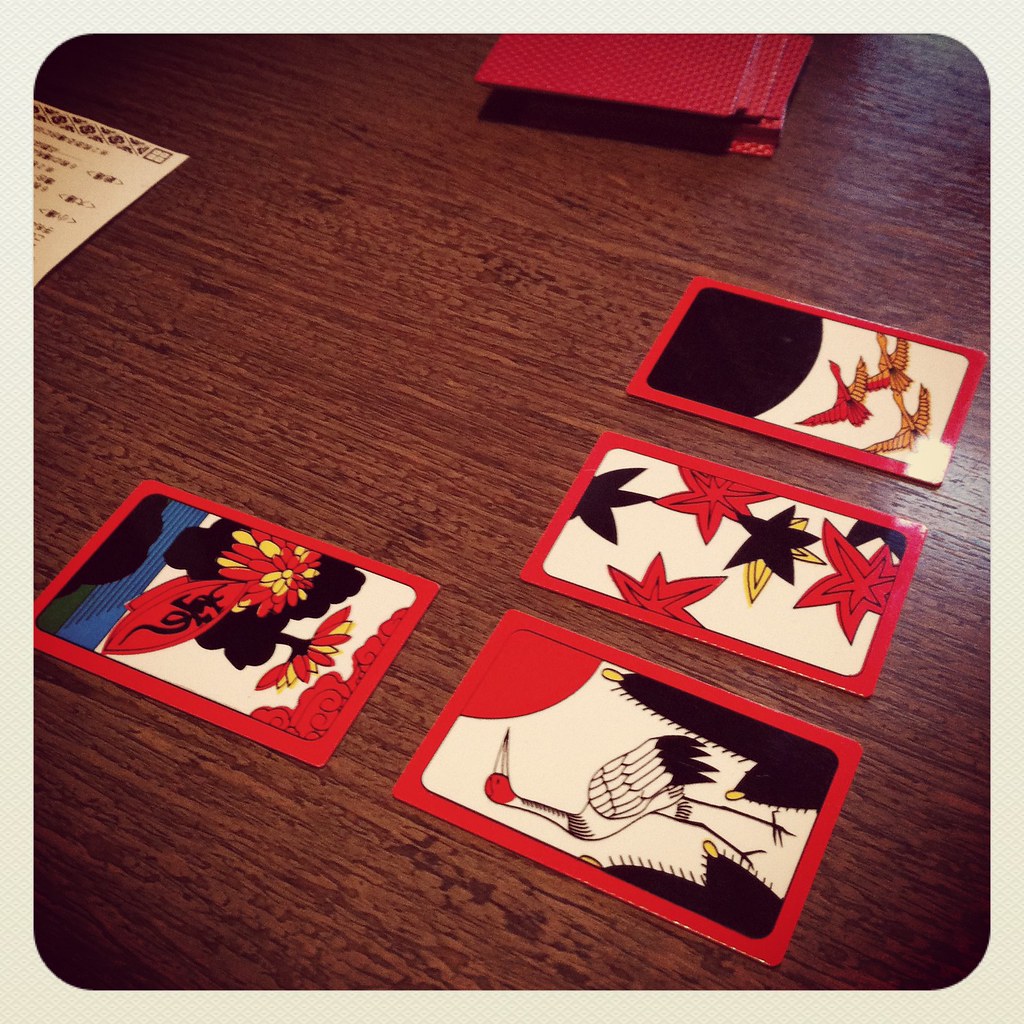The image captures a beautifully crafted table made of cherry wood, displaying a rich reddish hue that highlights the intricate grain patterns of the natural material. Atop the table rests a book with a deep red cover, accentuated by a ribbon running down its front, suggesting it might be a journal or a special edition book. Spread around the book are four distinct cards, each with unique designs and features.

The first card, which has a red border, depicts various geese in flight. One goose is predominantly red with a single golden wing, while two others are entirely golden. Notably, this card has a small tear in one corner, missing a piece of its red border.

The second card also features a red border and presents a simple, yet vibrant, design of scattered stars in red, black, and yellow on a white background.

The third card showcases a detailed drawing of a peacock with a red head and a long beak. Surrounding the peacock are cactus illustrations on either side and a half-moon arc shaded in red.

The final card is upside down and reveals an image of two flowers, adorned in red and yellow, accompanied by a red leaf upon which a tiny salamander rests. Behind this botanical scene, a tree is visible with a backdrop of what appears to be blue water. The intricate details and rich colors of the cards juxtapose elegantly against the warm tones of the cherry wood table.